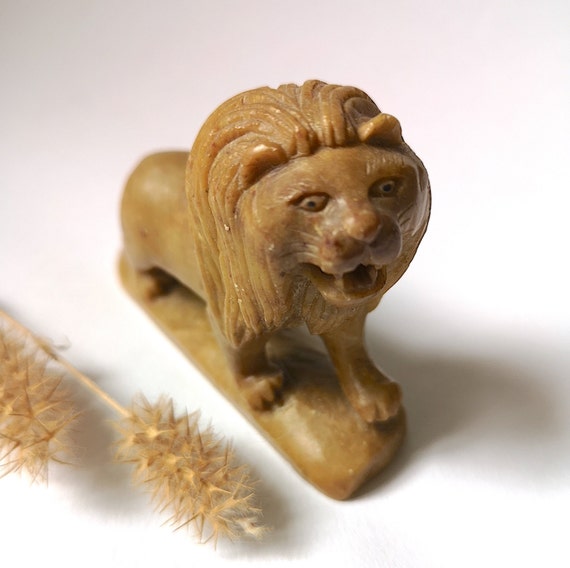A detailed close-up image features a detailed carving of a lion, seemingly crafted from a glossy, soft brown material, possibly soap, marble, wax, or clay. The lion is depicted in a side view with its mouth open, revealing two sharp fangs, and has a large, intricately detailed mane. Its eyes appear quite expressive, with one gazing straight ahead and the other slightly off to the side. This gives the lion a somewhat quirky, intense look. The figure is positioned on a white surface, with a background gradient from glary white at the bottom to light blue at the top. In the lower left corner of the image, there are two slender, tan stems resembling wheat stalks or brown mascara wands, topped with fuzzy, cotton-like tufts. These stalks protrude downward towards the image's center, casting delicate shadows to the right.